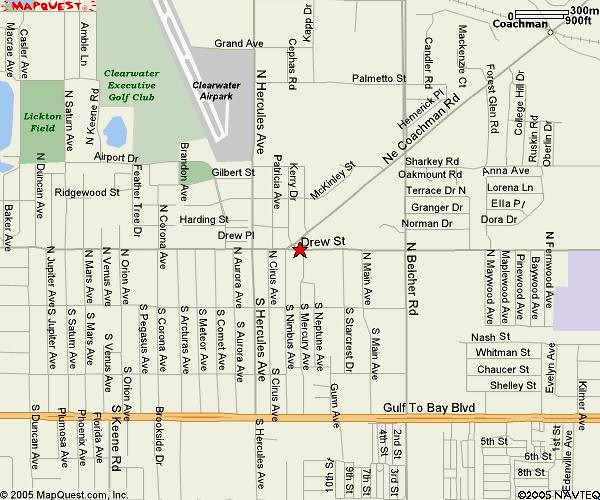The image is a detailed screenshot from MapQuest, showcasing a map centered on Drew Street, marked by a small red star in the middle. The map features various intersecting streets, named in black text, including McKinney Street, Glen Avenue, and Harding Street. Prominent thoroughfares like Gulf to Bay Boulevard, running horizontally near the bottom in dark orange, and Northeast Coachman Road are also visible.

At the top left corner, the MapQuest logo appears in red. Adjacent to Drew Street, several landmarks are highlighted: Licton Field (labeled in a light green background with green text), Clearwater Executive Golf Club (in dark green text on a green background), and Clearwater Airport (featuring a white airstrip and a dark gray field). To the top right, a legend indicates distance measurements with "300 M" and "900 FT" beside horizontal bars.

The map's background is predominantly cream-colored with detailed notations for streets and landmarks. Additionally, the bottom left corner contains the copyright notice "2005 MapQuest.com Inc.," and the bottom right adds "2005 Navtech," both in small text.